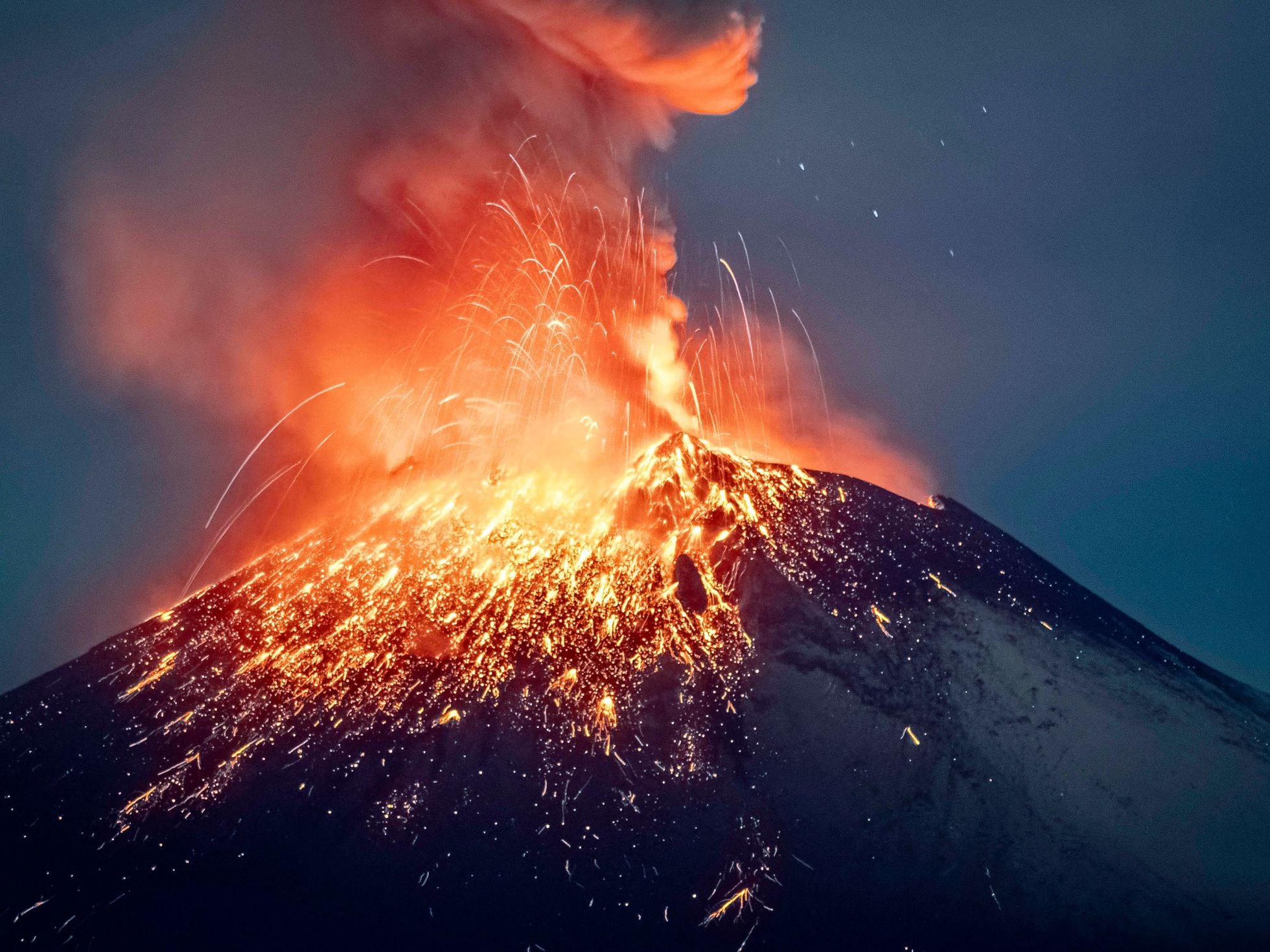This image depicts a nighttime volcanic eruption, ostensibly captured in a large square, computer-generated picture. Dominating the center of the frame, the volcano's apex extends downward towards the bottom left and right corners, shrouded in a charcoal and black landscape. The eruption scene is punctuated by bright white and orange specks resembling embers and lava. Streaks of fiery lava ascend vertically, resembling fireworks, while a thick billow of orange-gray smoke clouds the view overhead. The dark bluish-gray sky is visible in the background, flecked with what appear to be small white ashes or stars, enhancing the dramatic nocturnal setting.